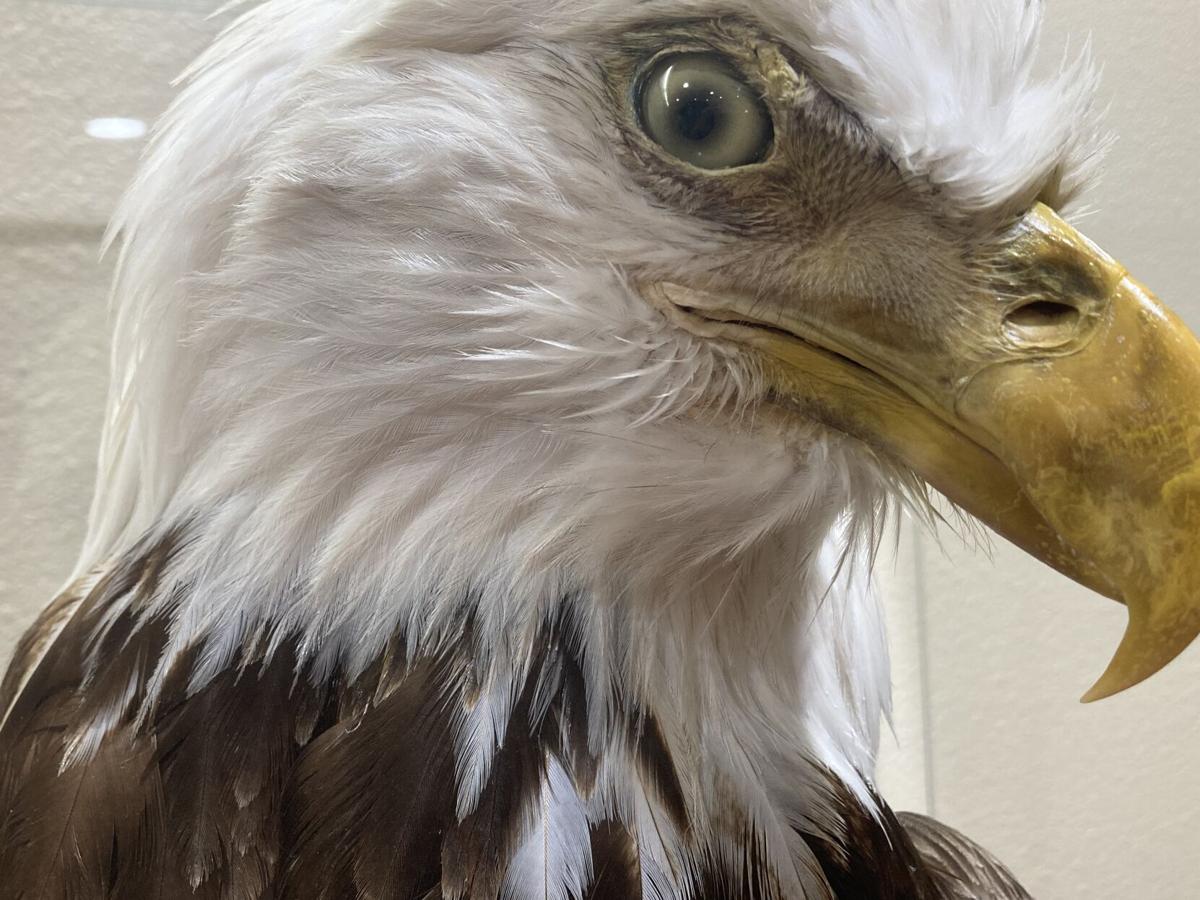A highly detailed close-up image of an American bald eagle's head, with a sharp focus on its menacing expression. The eagle’s eyes are especially captivating, featuring a pale green, glazed-over iris with a black pupil, capturing reflections that add depth and realism. Its large, curved beak is a striking yellowish-gold, contrasting starkly with the white feathers that adorn its head. The intricate pattern of the feathers is clearly visible, from the dark brown ones at the bottom, near the shoulder and belly area, blending into the white plumage covering the neck and head. The background reveals a somewhat ambiguous setting with white brick walls and plain white surfaces, suggesting the possibility that the eagle might be either a very realistic replica or a meticulously preserved taxidermy specimen, although the naturalistic details lend credence to its lifelike appearance.